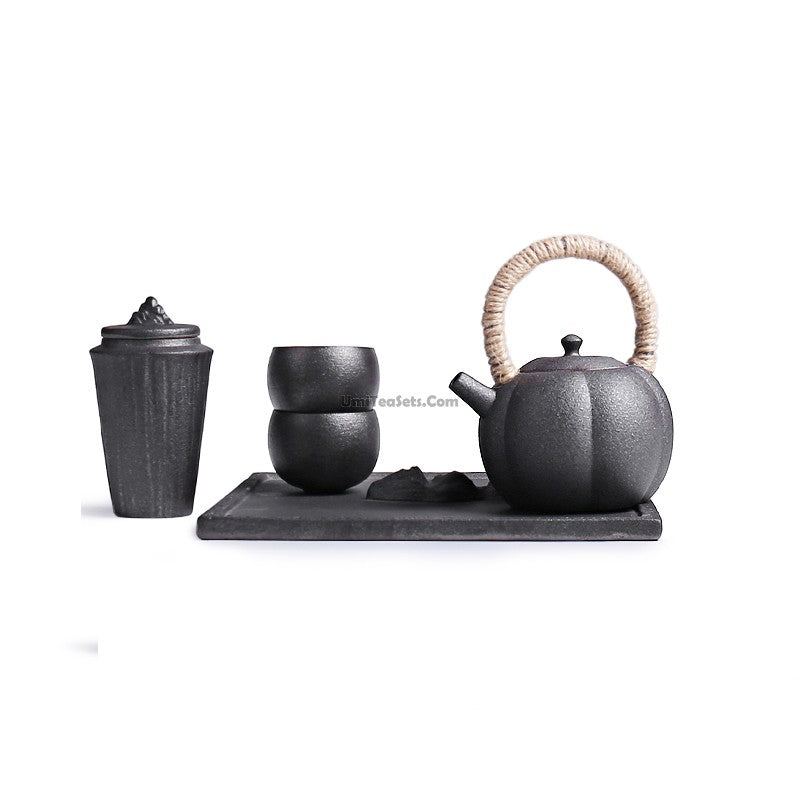The image depicts an elegant black tea set presented on a black serving tray against a white background. The set includes two spherical black stone cups with their tops cut off, stacked on the left side of the tray. The centerpiece is a black teapot, which is pumpkin-shaped with distinct ridges, featuring a short spout and a handle wrapped in rope or twine for an artisanal touch. Off to the left of the tray, there's a black stone shaker cup with a lid. A watermark reading "umitesets.com" appears across the middle of the image, reinforcing the tea set theme amidst the monochromatic design.